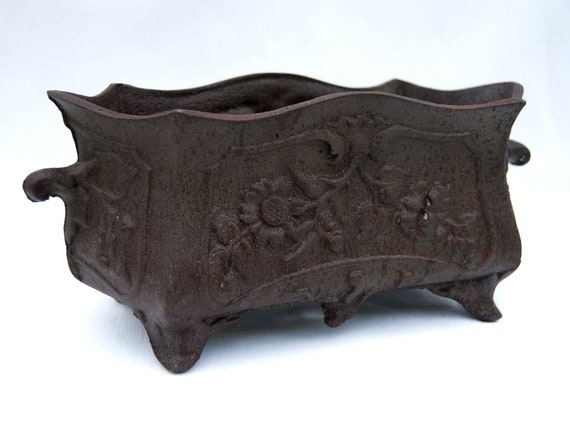The image features an ancient-looking rectangular container, potentially an artifact of European or colonial origin. This box-like vessel is displayed in a white room on a white surface, with a background that gradually fades to a grayish light blue near the top. The container itself is aged and dirty, exhibiting a reddish-brown hue, possibly from rust or dirt. The open-faced container has wavy top edges and intricate engravings of flowers within rectangular raised lips on its sides. There are handles protruding on either of the shorter sides. Detailed claw-like feet are situated at each corner, with stabilizing feet in the center of the longer sides. The photo captures it from an angle looking towards the front right-hand side, with the back right-hand side angled away toward the background.